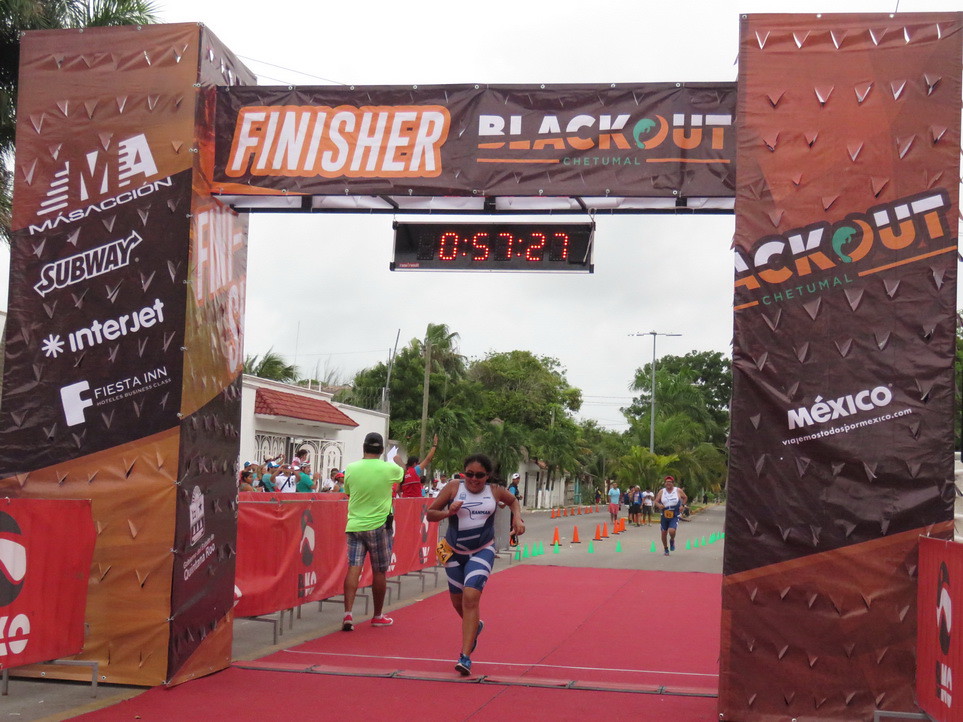In this photograph, a female runner in a white and blue running suit, with blue sneakers, is crossing the finish line of a marathon. Behind her, another runner is swiftly approaching. The finish line consists of a large archway, draped with tarpaulins bearing the names of sponsors such as Subway, Interjet, and Fiesta Inn, indicative of the event being held in Mexico. The horizontal bar of the arch above the runner displays the word "Finisher" and below it is a digital timer showing "57:27." To the left of the finish line stands a man with his back to the camera, and in the far distance, more runners can be seen on the path. The race route is marked by red and green traffic cones, guiding the participants towards the end. Adding to the festive atmosphere, a red carpet covers the ground at the finish line.